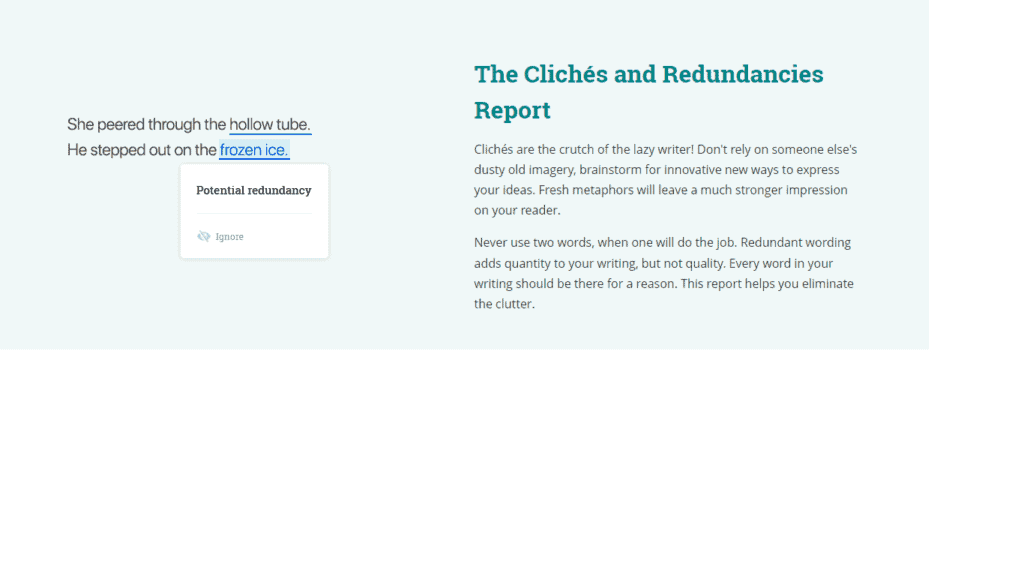This image captures the "Clichés and Redundancies Report," showcasing an analysis tool designed to help writers identify and eliminate unnecessary verbiage. On the left side of the report, examples of redundant phrases are presented: "She peered through the hollow tube" and "He stepped out on the frozen ice." Both phrases underline the redundant words—'hollow' in conjunction with 'tube' and 'frozen' with 'ice'—highlighting the overuse of descriptors that do not add value. The report emphasizes avoiding clichés and redundancies as they can dilute the quality of writing. By brainstorming original metaphors and ensuring each word serves a purpose, writers can create more impactful and concise prose. Helpful features include an option to ignore specific suggestions if deemed necessary. The detailed guidance underscores that every word should contribute meaningfully, steering writers away from reliance on worn-out imagery and redundant phrasing to foster more evocative and articulate expression.